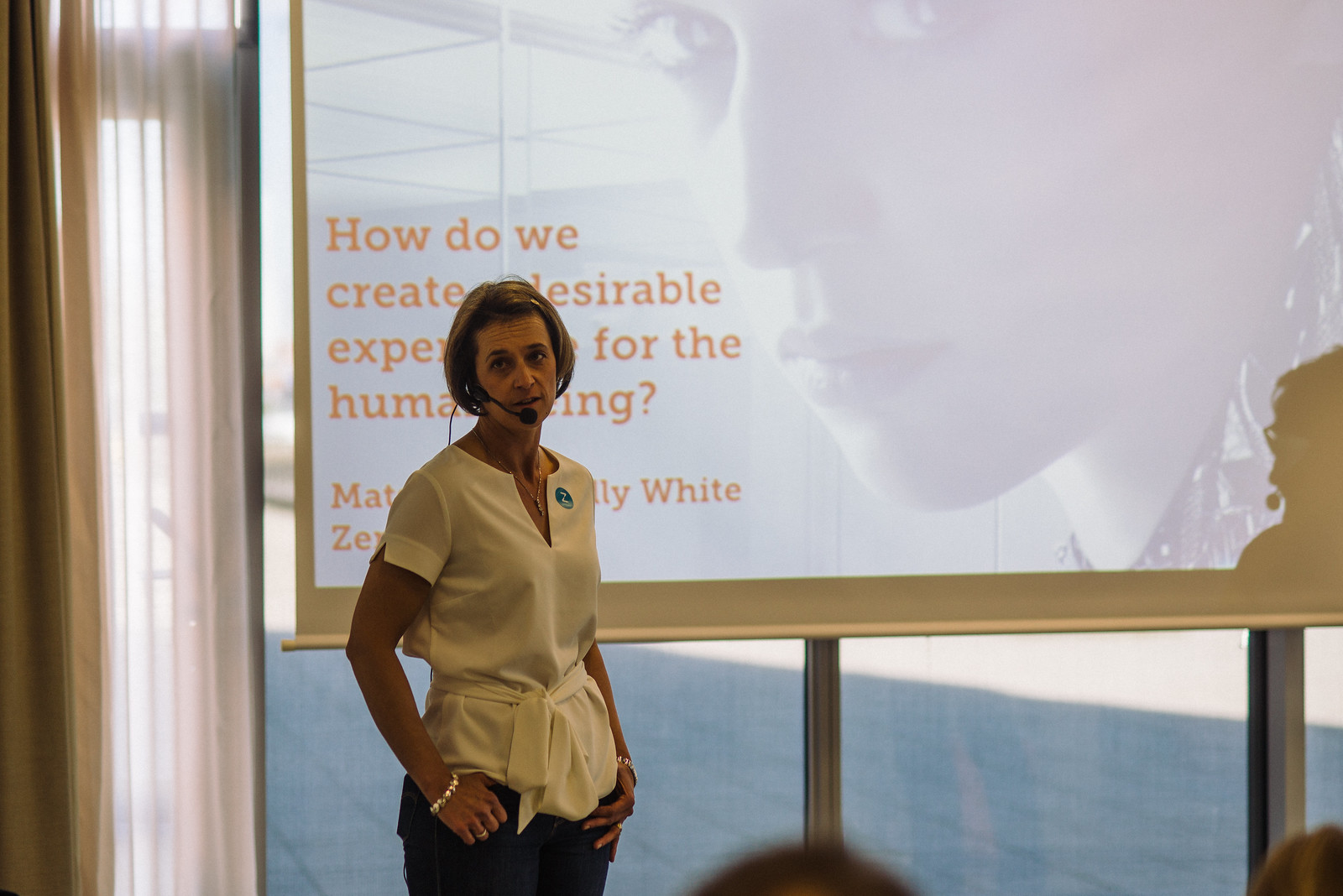The image captures a woman, who appears to be the main focal point, likely taken during an indoor presentation or conference. She stands facing the right side of the image with her head turned towards the camera. She has short blonde hair and wears a white shirt with a sticker on the left side, paired with dark trousers. The shirt is tied around her waist, and she also sports a headset with a microphone, suggesting she is speaking or presenting. She accessorizes with a watch or bracelet on both wrists and has a handkerchief on her hips. Her expression is one of visible displeasure or disgust.

In the background, there is a projection of a translucent image of a younger girl, presenting a somewhat ghostly appearance. The projection displays an incomplete text due to the woman partially blocking it, reading: "how do we create desirable expectations for the human being?" Some of the author’s name is obscured by the woman. On the left side of the picture, you can see a window with translucent curtains, and on the right, the shadow of an object or person appears. Additionally, the tops of two audience members' heads are visible, indicating the presence of a small crowd.